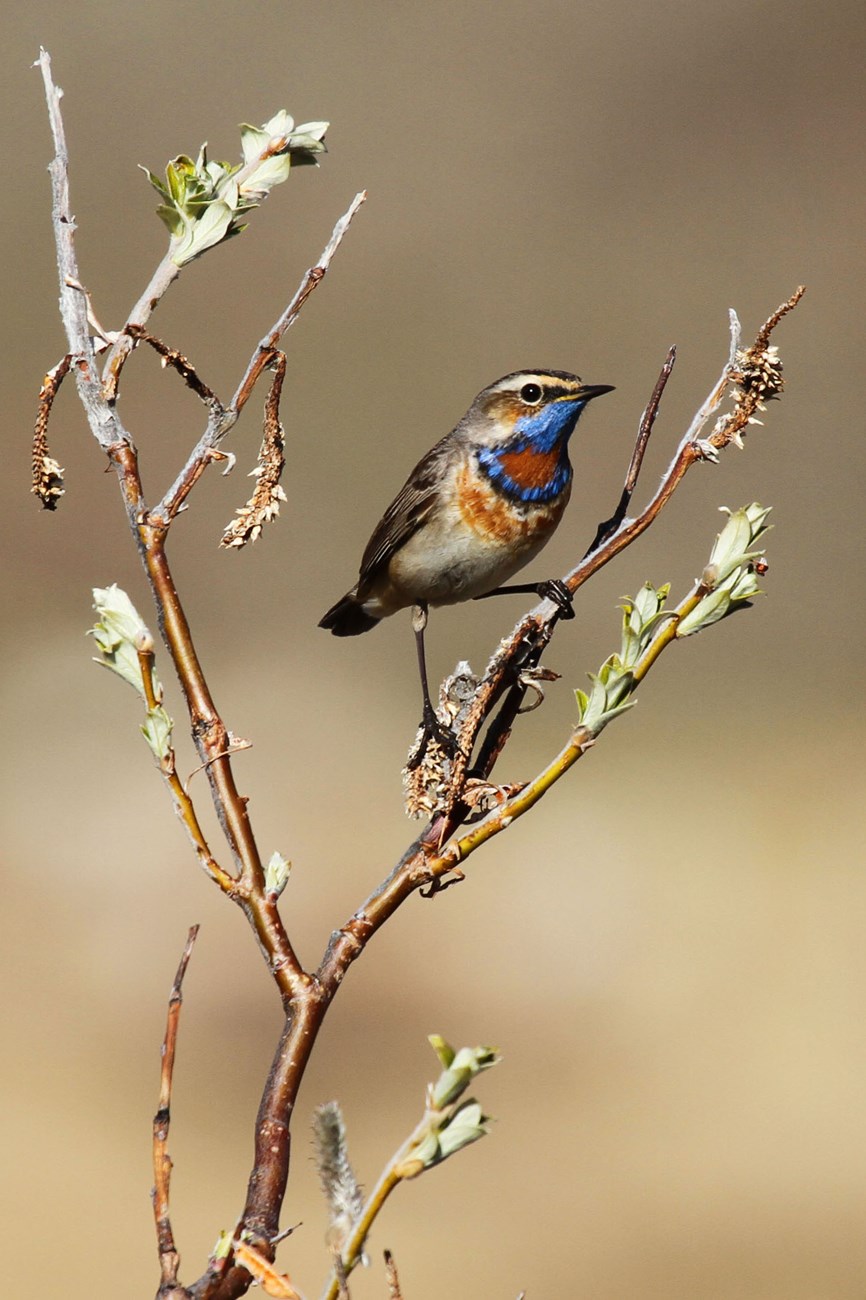This vivid photograph captures a small, ping-pong ball-sized finch perched on a barren brown twig that dominates the frame, extending vertically through the image. The twig, adorned with both green buds just about to bloom and old brown seeds, is the only element other than the bird and the blurred background of mixed brown, gray, tan, and off-white hues. The finch is perched on the top right of the twig, gripping it with its thin, black legs and feet. The bird's plumage features a predominantly brown back and a lighter, whitish-brown underbelly. Its breast is gold, transitioning to a beige stomach. Its throat is striking with cascading shades of vibrant blue, red, orange, and black. The bird’s small, sharp beak and single visible black eye, accentuated by a lighter brown blaze above it, enhance its alert expression as it leans slightly forward, possibly poised for flight.